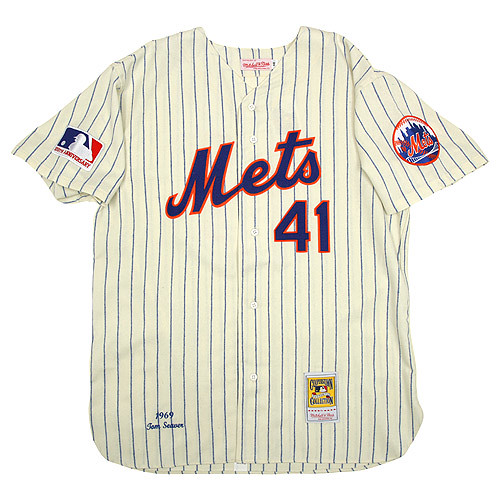The image features a vintage Mets baseball jersey set against a plain white background. The jersey is short-sleeved and button-down, with a rounded hemline. Its color is a creamish-tan, resembling an aged white, adorned with vertical blue pinstripes. Across the chest, "Mets" is prominently printed in dark blue cursive letters, outlined in orange. Just below the lettering, positioned off-center towards the right, is the number 41, also in dark blue with an orange trim. On the right sleeve is a circular Mets logo, depicted as a baseball with an orange rim. The logo includes a blue cityscape backdrop with "Mets" written in orange cursive across it. The left sleeve features the Major League Baseball logo, displaying a player hitting a ball, in the traditional colors of white, blue, and red. At the bottom left of the jersey, the year "1969" is inscribed along with a name, and there's a small gold badge on the bottom right.